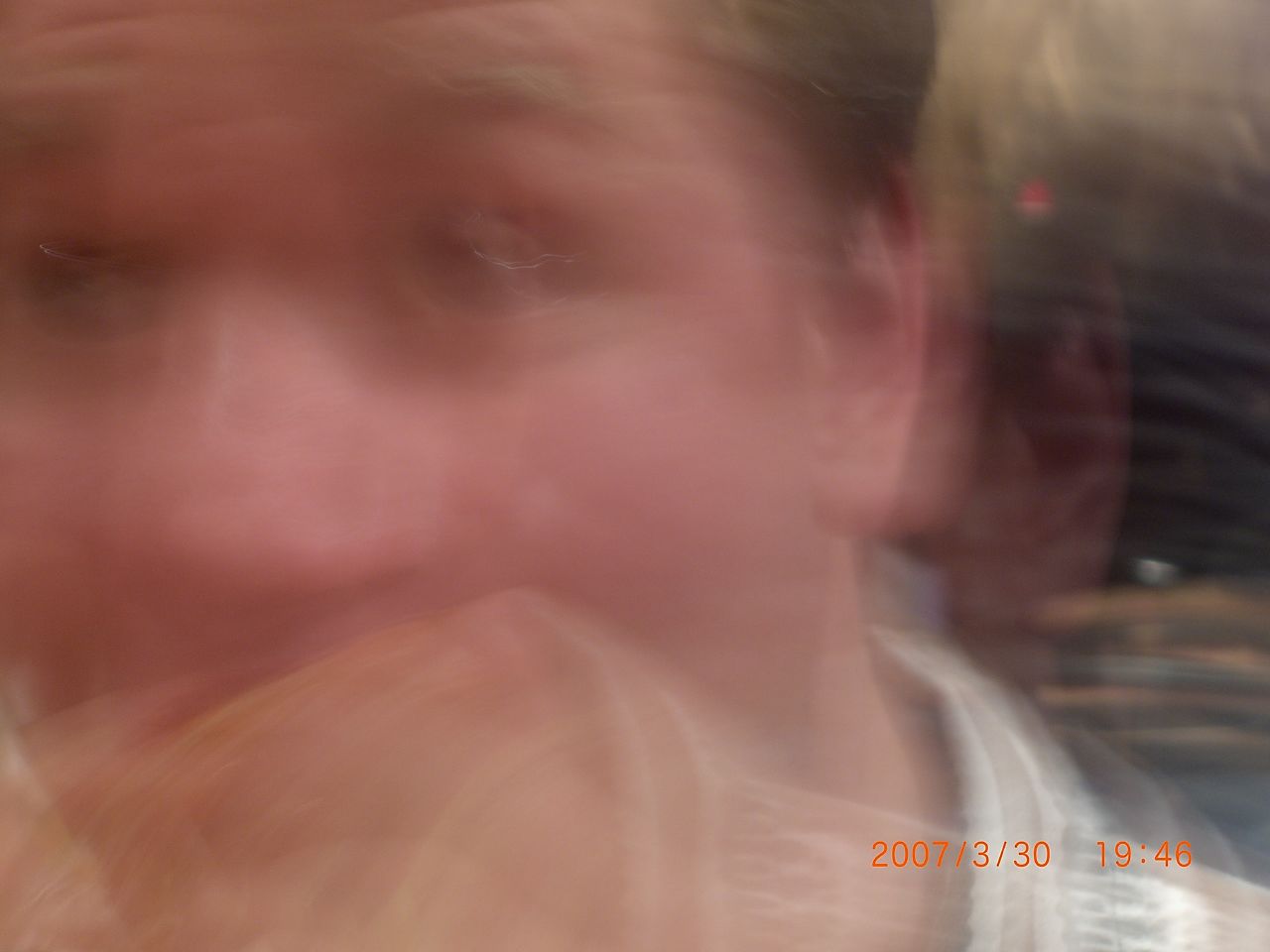This photograph is highly blurry and features the face of a human subject. The lower portion of the face, from the lips downward, is obscured by an indistinguishable object due to the image's poor quality. The person appears to have light skin, dark-colored eyes, and possibly short, dark hair, suggesting it is likely a man's face. The individual is dressed in a light-colored shirt. At the bottom right corner, there is an orange timestamp that reads "2007 3 30 at 19:46." The background behind the person is predominantly dark, with scattered patches of red, white, green, beige or brown, and perhaps some silver, although the exact details are difficult to discern due to the image's blurriness.